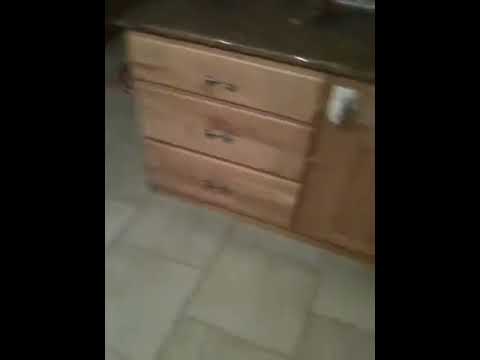This image features a very blurry photograph of a cabinet or stand with a hard, shiny surface, possibly made of stone or marble. The stand, located to the top right of the image, has a dark-colored countertop and three light brown wooden drawers, each equipped with a handle. Next to the top drawer is something white, but its blurriness makes it indiscernible. On the countertop, there is a small, possibly black object that could be a remote control; however, the blur obscures its precise identification. The floor in the image is tiled and gray in color, filling the bottom left portion of the scene. The photo appears to be taken indoors, likely in a kitchen area, from a downward angle, capturing a close-up that showcases the texture and color contrasts within the space. The overall color palette includes shades of black, gray, brown, and white, though the image lacks any text or words to provide additional context.